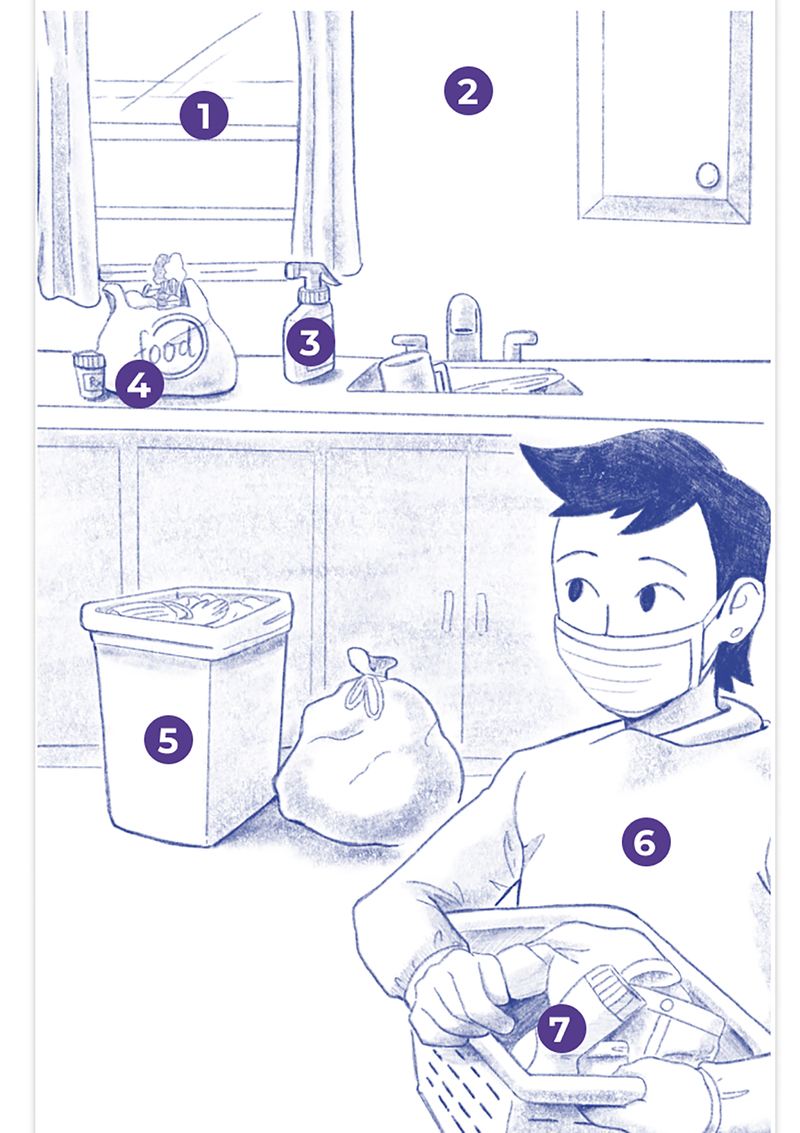This is a hand-drawn illustration done in blue pen, with white used for negative space, featuring a detailed depiction of a kitchen scene. The image is in portrait orientation and focuses on a young boy with long black hair, wearing a mask, standing on the bottom right corner. He is holding a basket of laundry and is pictured from head to mid-waist, facing the viewer, but looking up towards the top left corner of the image. 

The kitchen is intricately detailed, indicating different numbered objects, each surrounded by a black circle with white text numbering 1 through 7. The numbers and their corresponding objects are as follows:
1. The window above the kitchen counter, located at the top left.
2. The wall space to the right of the window.
3. A spray bottle (possibly Windex) located on the counter below the window.
4. A bag of groceries labeled "Food" positioned on the counter at the top left.
5. A trash can found further down the left side of the image.
6. The boy's hoodie or sweatshirt, with the number marked on his chest.
7. The basket of laundry carried in the boy's hands at the bottom right.

Adding to the depth of the illustration, the counters and cabinets in the upper right corner, and the detailed kitchen items further enhance the scene's realism, creating a comprehensive and vivid depiction of the boy's kitchen interior.